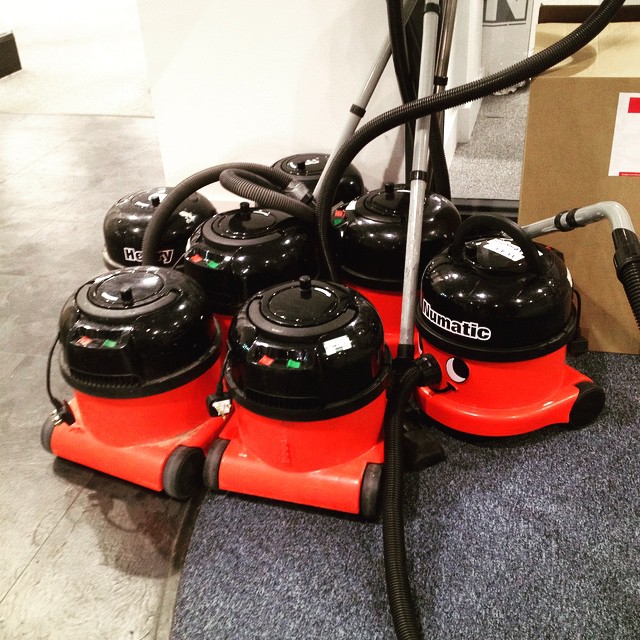The image depicts a group of seven bright red shop vacuums, each characterized by a black lid with green and red switches, and mounted on two black rubber wheels. They are huddled together in an indoor space, which features a gray concrete ground on the left and bluish-gray carpet on the right, with a white wall and a cardboard box in the background. The vacuums have a distinct curved shape at the front, resembling an upside-down Tupperware container. Notably, one of the vacuums is facing forward, displaying cartoonish eyes, a black smiley face, and a long "nose" formed by the hose adapter, evoking a humorous appearance. These vacuums, often associated with the classic red designs featuring googly eyes, have their extension hoses and tubes extending upward and towards the right, some connecting to metallic cylinders. All of their power cables are unplugged and hang loosely.